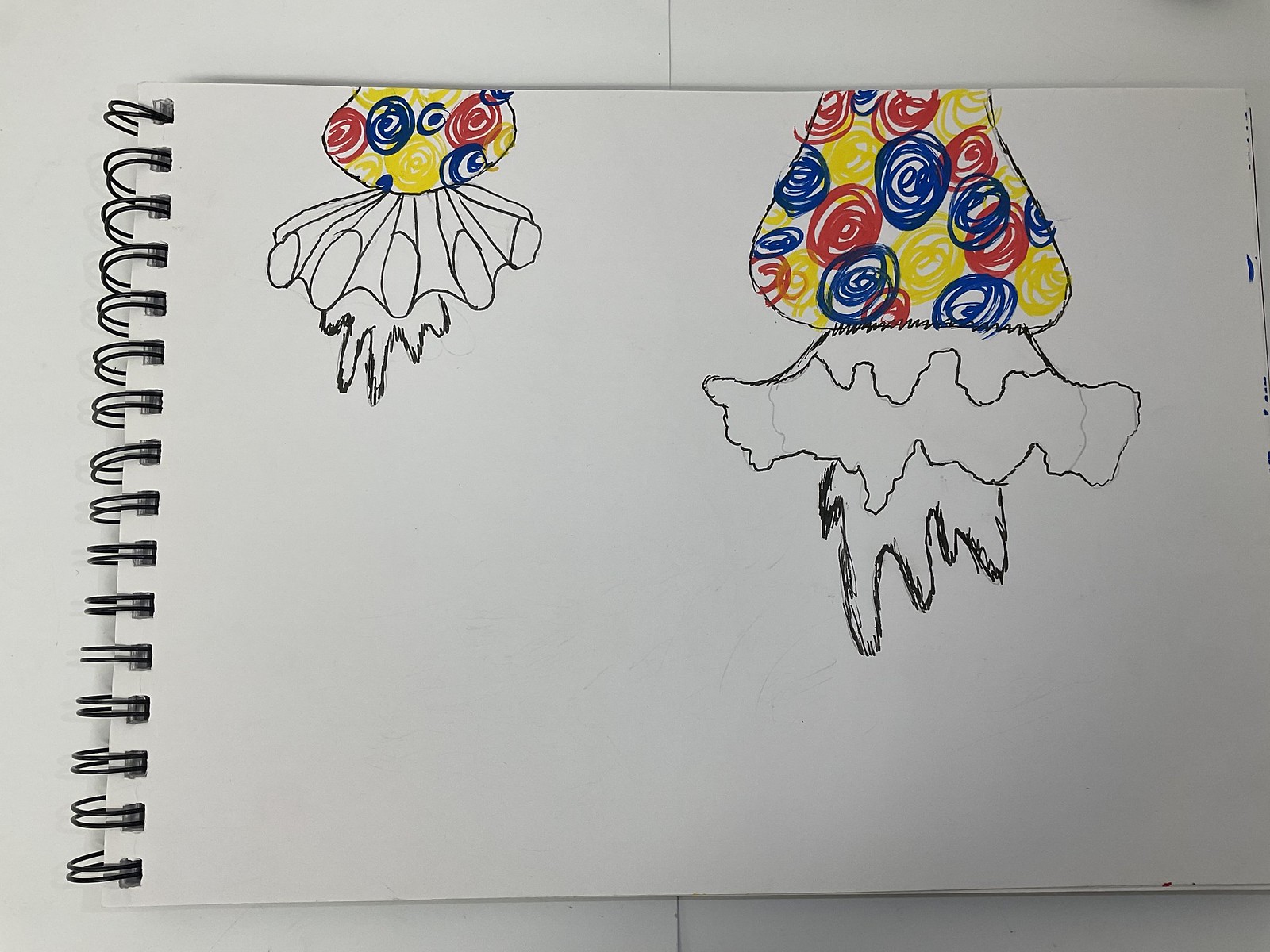The image depicts a wire-bound notebook, featuring double metal rings along its left spine. The pages are unlined and contain detailed drawings. The illustrations focus solely on the wrists and hands protruding from elaborately decorated sleeves. The sleeves are adorned with yellow, red, and blue circles, culminating in lace trims reminiscent of a clown's costume. The hands extend gracefully from these ornate cuffs, adding an intriguing element to the composition.